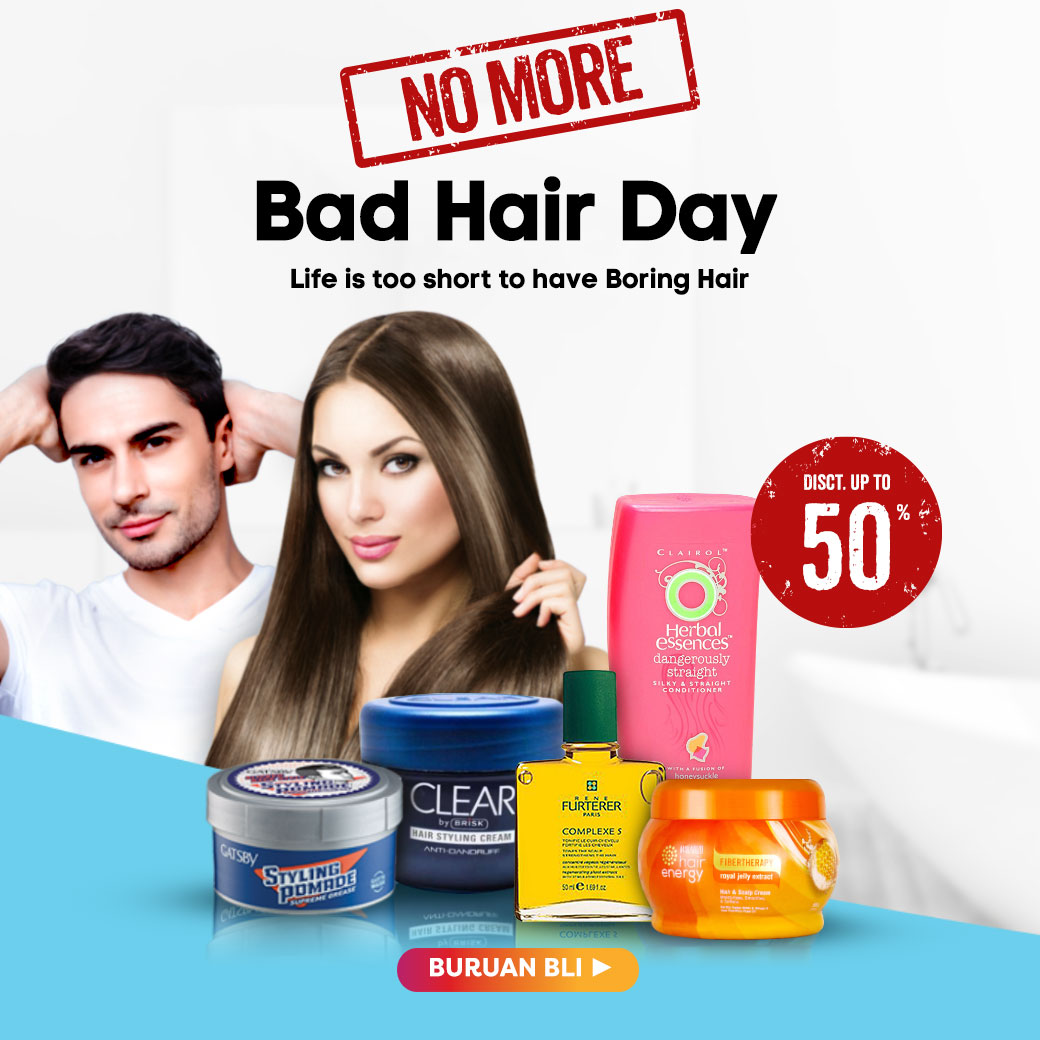The advertisement features a vivid layout aimed at promoting various hair styling products. At the top, the ad prominently displays a bold red box with the text "NO MORE" in red letters. Just below this, in bold black letters, it states "Bad Hair Day" followed by a smaller black sentence that reads, "Life is too short to have boring hair." The image includes two models: a light-skinned man with dark hair, wearing a white V-neck shirt, and a light-skinned woman with dark brown hair and prominent makeup, gazing directly at the camera. The bottom part of the advertisement showcases an assortment of colorful hair products—cylinders and jars in hues of blue, gray, orange, pink, and yellow—arranged on an angled light blue stripe. To the right of these products, there is a red circle containing the text "D-I-S-C-T up to 50% off" in white letters. At the bottom of the image, an orange-to-red gradient banner features a button labeled "Buron Blea" with an arrow pointing to the right, adding a call to action.